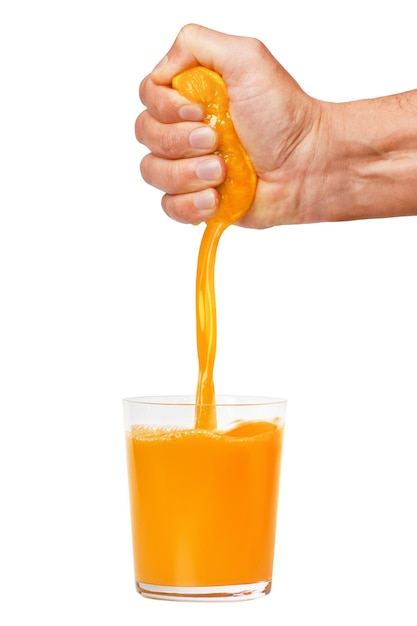The image depicts a light-skinned hand, likely that of a Caucasian male, squeezing juice from an orange half into a nearly full, short clear glass cup. The liquid flowing from the orange appears unnaturally thick and concentrated, almost as if it were manufactured juice. The scene is superimposed onto a stark white background, giving an impression that the glass is floating in midair. The overall quality of the image is very clear and brightly lit, with the orange and juice prominently colored in vivid orange, creating a strong visual contrast against the otherwise minimalist setting.